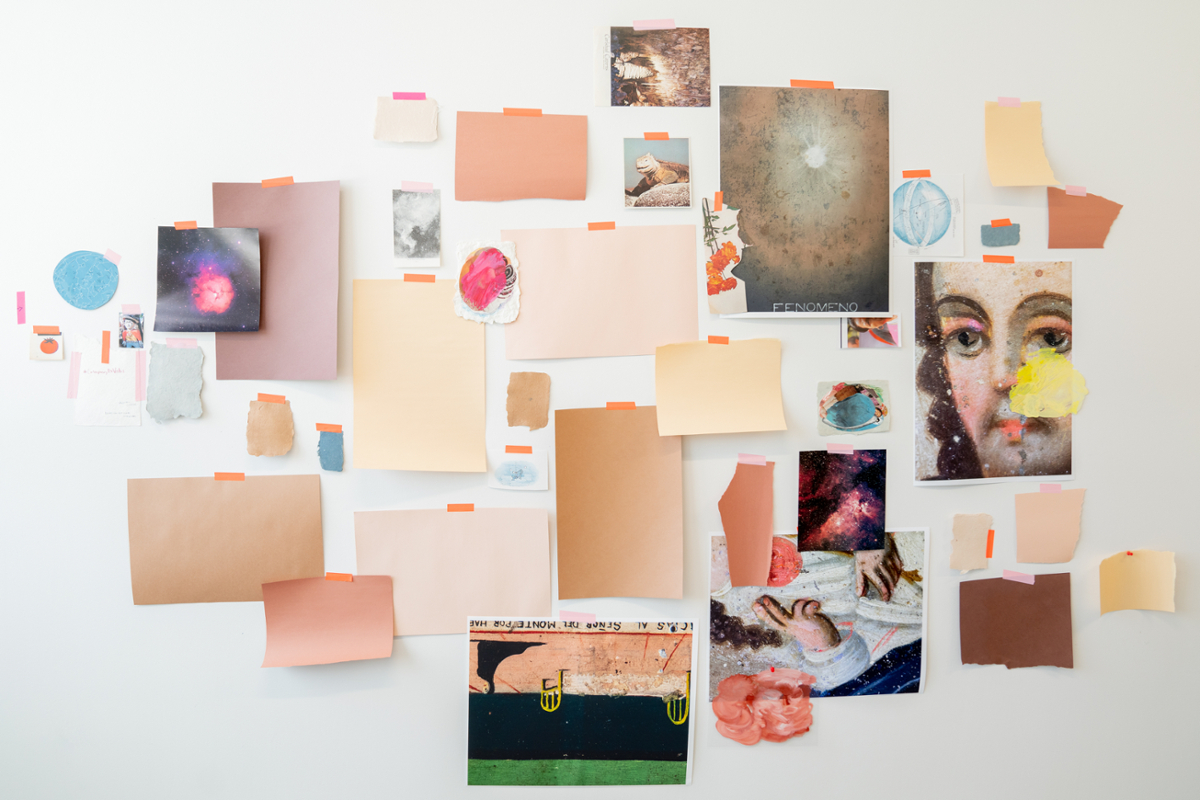This photo showcases a vibrant collage of various pieces of construction paper and artwork meticulously taped onto a stark white wall. The myriad sheets of paper include an array of pastel shades such as tan, pink, beige, mauve, and apricot, with occasional accents of blue and green. These papers, some blank and others featuring prints or paintings, are arranged in a mix of horizontal and vertical orientations, creating a visually dynamic and abstract design. Interspersed among these are intriguing images: a close-up of a stone figure’s face, a hand gesturing with two fingers up, a fiery meteor, celestial space scenes, and possibly an iconic figure like Shakespeare or a saint. The collage utilizes vivid fluorescent orange and pink tape for securing the pieces, adding to the overall eclectic and warm-toned aesthetic. Each element varies in shape and size—ranging from small squares and large rectangles to circles—culminating in a visually captivating and richly detailed montage.